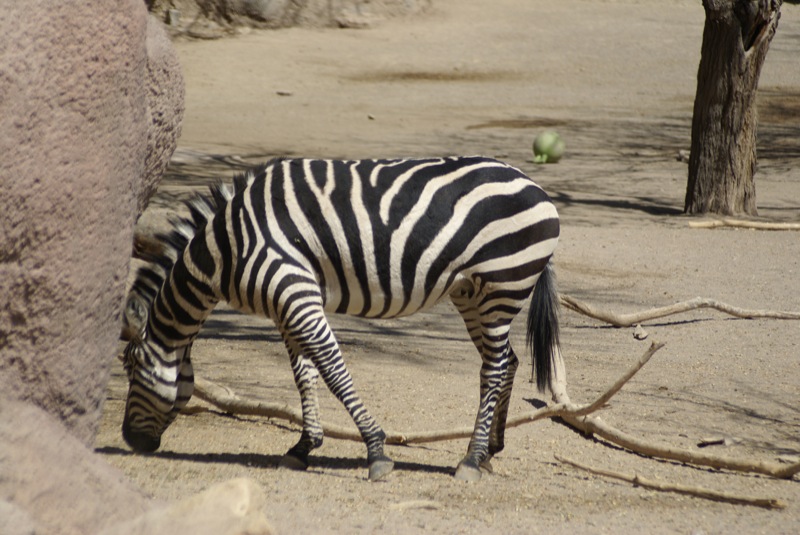In this detailed image, a zebra, distinguished by its signature black and white stripes, stands in the center on a flat, barren expanse of dry dirt with no grass in sight. The zebra, resembling a horse with hooves, a tail, and a head bent down, appears to be sniffing or searching for food on the ground. To its immediate left is a prominent rock, which is characterized by rounded and worn edges, suggesting it may have been placed deliberately, likely indicating a zoo or sanctuary setting rather than the wild. Strewn on either side of the zebra are several long, loose branches. Towards the upper right corner of the image, there's the trunk of a tree, and below it, a small green fruit or vegetable, possibly fallen from the tree, lies on the ground. The backdrop to the left shows additional rocky cliffs, further reinforcing the idea of an artificial habitat. The scene is unmistakably set outdoors during daylight, emphasizing the zebra's natural yet maintained environment.